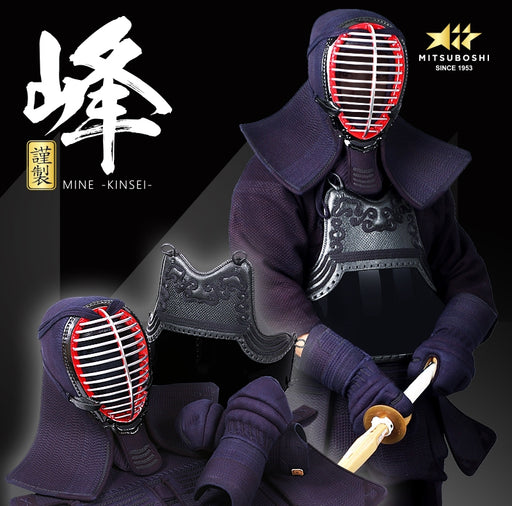The image features a Japanese-inspired fencing scene centered around an individual clad in full regalia. The person is fully covered in a purple cloak, with their head, chest, arms, legs, and hands all protected by the armor. Notably, the individual wears a metal fencing mask with a red rim, from which piercing eyes, and part of the nose and mouth, can be discerned upon closer inspection. The individual wields a practice sword, likely made of wood or plastic, with both hands gripping it firmly.

To the left of the person, a complete piece of the headgear, including the helmet and gloves, is displayed prominently. Further, the scene features a breastplate, adding to the detailed depiction of the armor. In the upper right corner is the logo of Mitsuboshi, a company established in 1953, recognizable by its three-star emblem. Adjacent to the logo, Japanese calligraphic writing reads "MINE-Kinsei," with some inscriptions set against a black background and others framed in a gold inset, adding an authentic touch to the image.

Overall, the photo captures a detailed and culturally rich representation of Japanese sword fighting armor, merging historical artistry with modern craftsmanship.